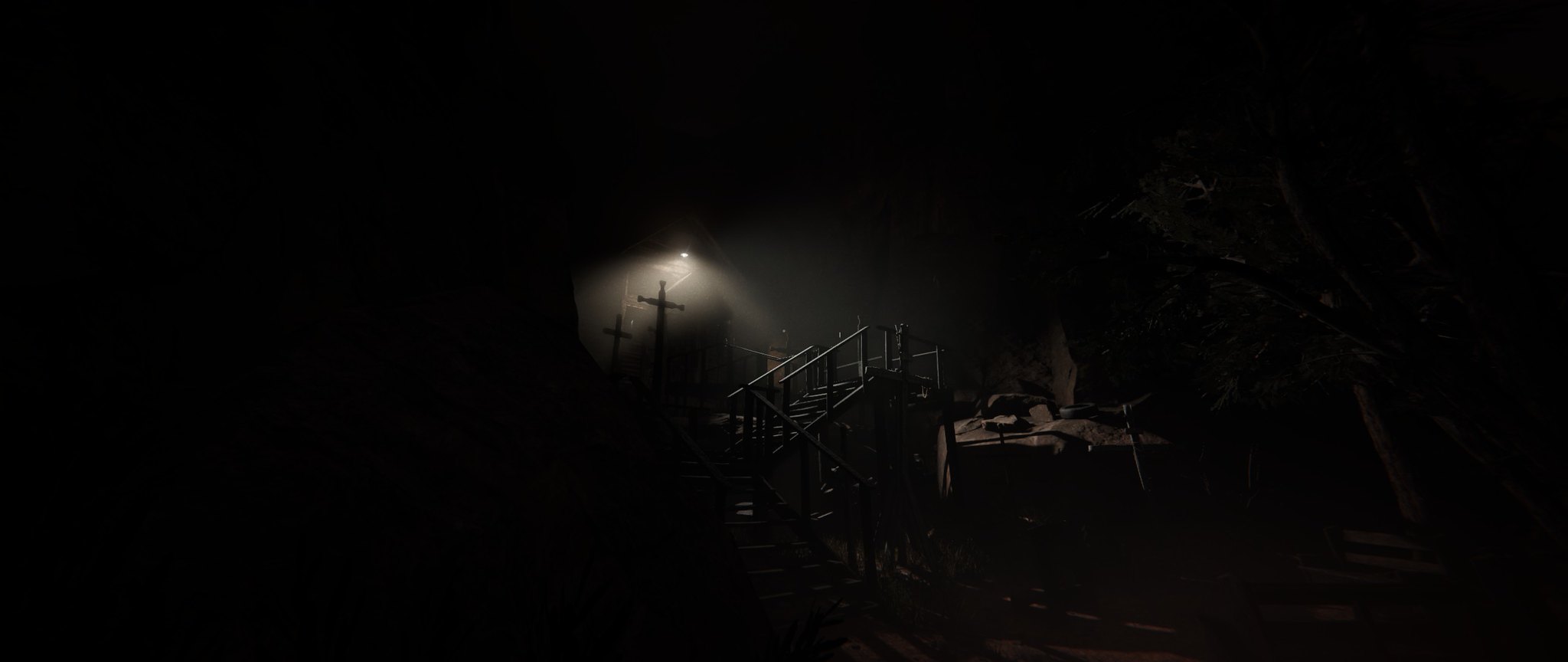A nighttime photograph or computer-generated image depicts an extraordinarily dark outdoor scene outside a building, making details difficult to discern. Wooden stairs lead up to the entrance of the building, suggesting a rustic or woodsy environment. Near the top of the stairs, crucifixes are visible, adding an eerie element to the setting. A solitary floodlight illuminates the area near the door, casting the only significant light. At the base of the stairs lies a decaying vehicle, adding to the post-apocalyptic atmosphere of the scene.